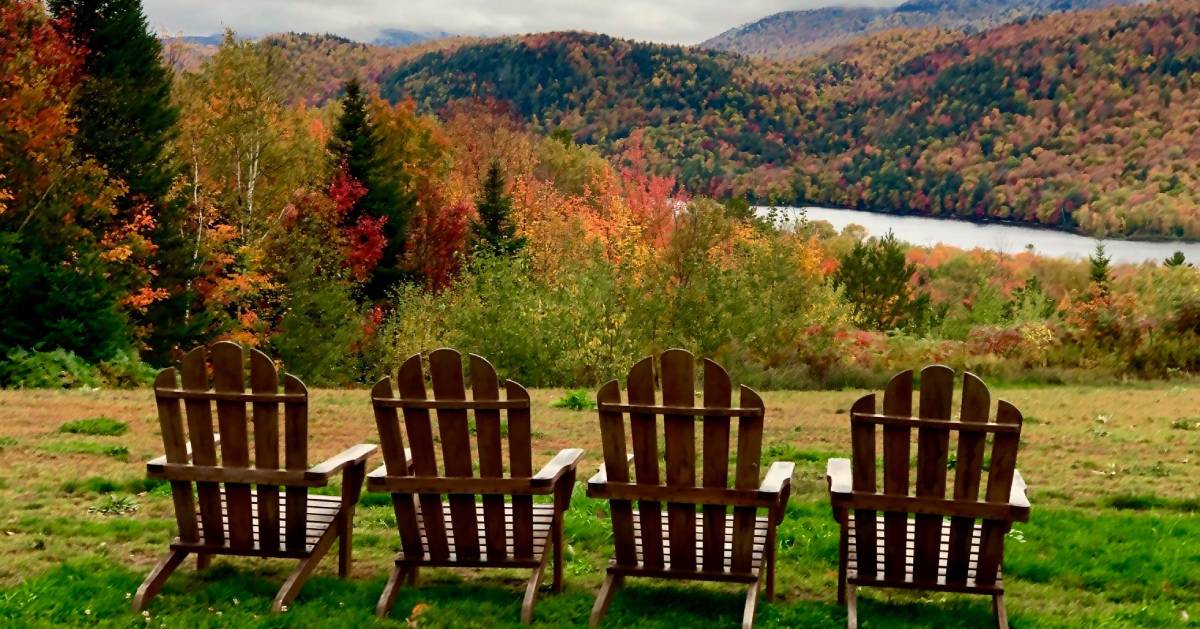In this vibrant outdoor scene, four neatly arranged wooden Adirondack chairs sit atop a grassy hill, facing a breathtaking panoramic view. Below lies a river that gracefully winds its way through the landscape, enhancing the picturesque setting with its gentle flow. In the background, an expansive tapestry of mountain ranges unfolds, blanketed in a rich palette of fall foliage. The trees, adorned in vivid hues of red, orange, yellow, and varying shades of green, signal the arrival of autumn. These colorful forests stretch up to the mountains, whose peaks are crowned with clouds under a slightly overcast but serene blue sky. The chairs, crafted from wood with five slats on the back and double armrests, are perfectly aligned, inviting viewers to sit and immerse themselves in the natural beauty.